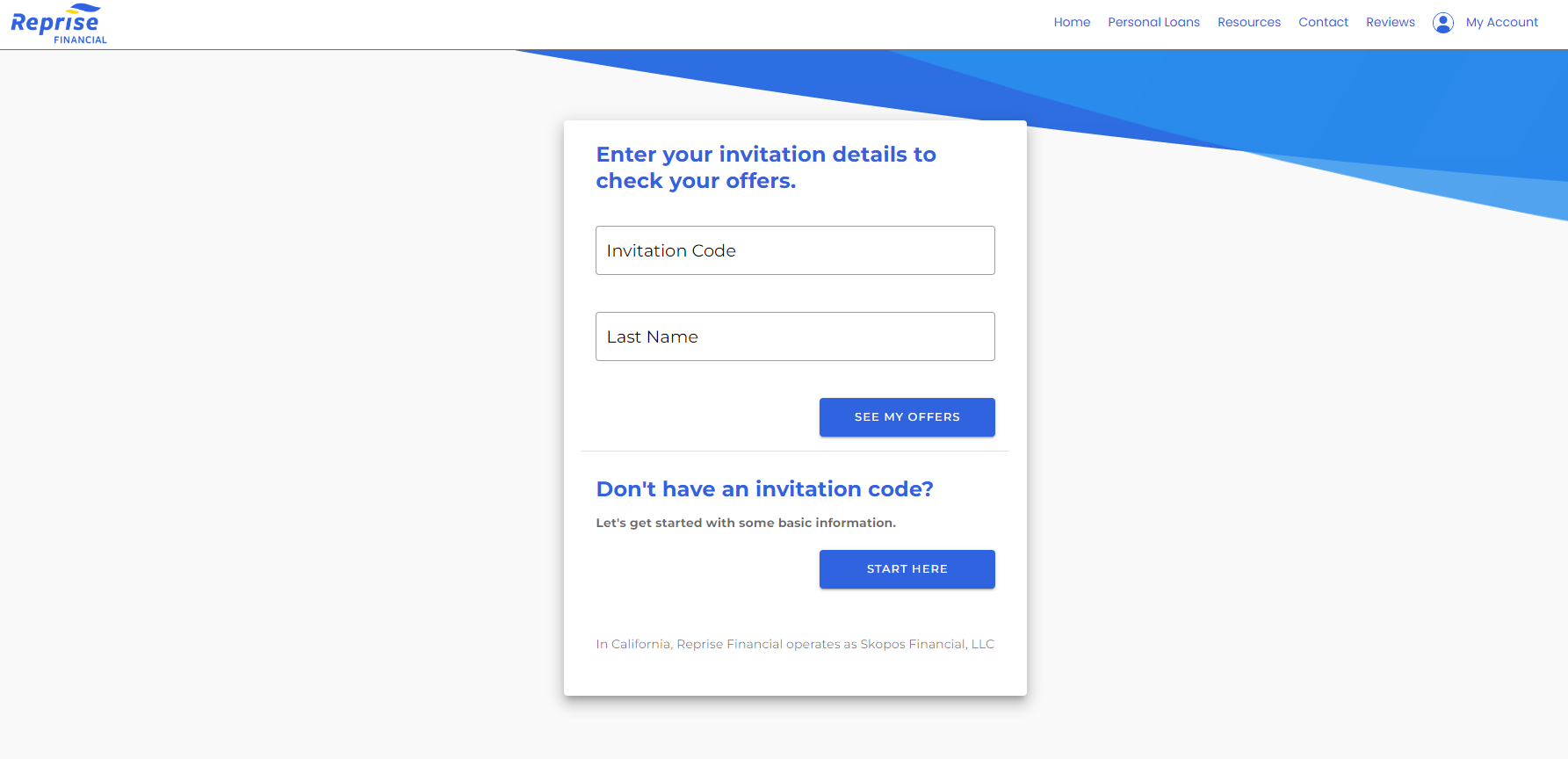The image depicts a webpage, which could belong either to a tablet or monitor screen, for an entity named Reprise. The webpage appears to be associated with a car dealership or a loan company, possibly identified as Reprise Financial. The user is already logged in, as indicated by "My Account" located at the upper right corner of the page. The page predominately features blue and white hues, with lettering in blue, and a background in a light beige-gray color. A popup dialog box in white is prominently displayed, prompting the user to enter an invitation code and their last name to access personalized offers. An option to proceed without an invitation code is also available, indicated by the text "Don't have an invitation code, start here."

The navigation menu at the top comprises several options: "Home," "Personal Loans," "Resources or Refinancing," "Contact," and "My Account." A small, blue triangular design element appears at the upper right corner of the screen. The overall design maintains a clean and minimalistic aesthetic, utilizing primarily blue and white colors.